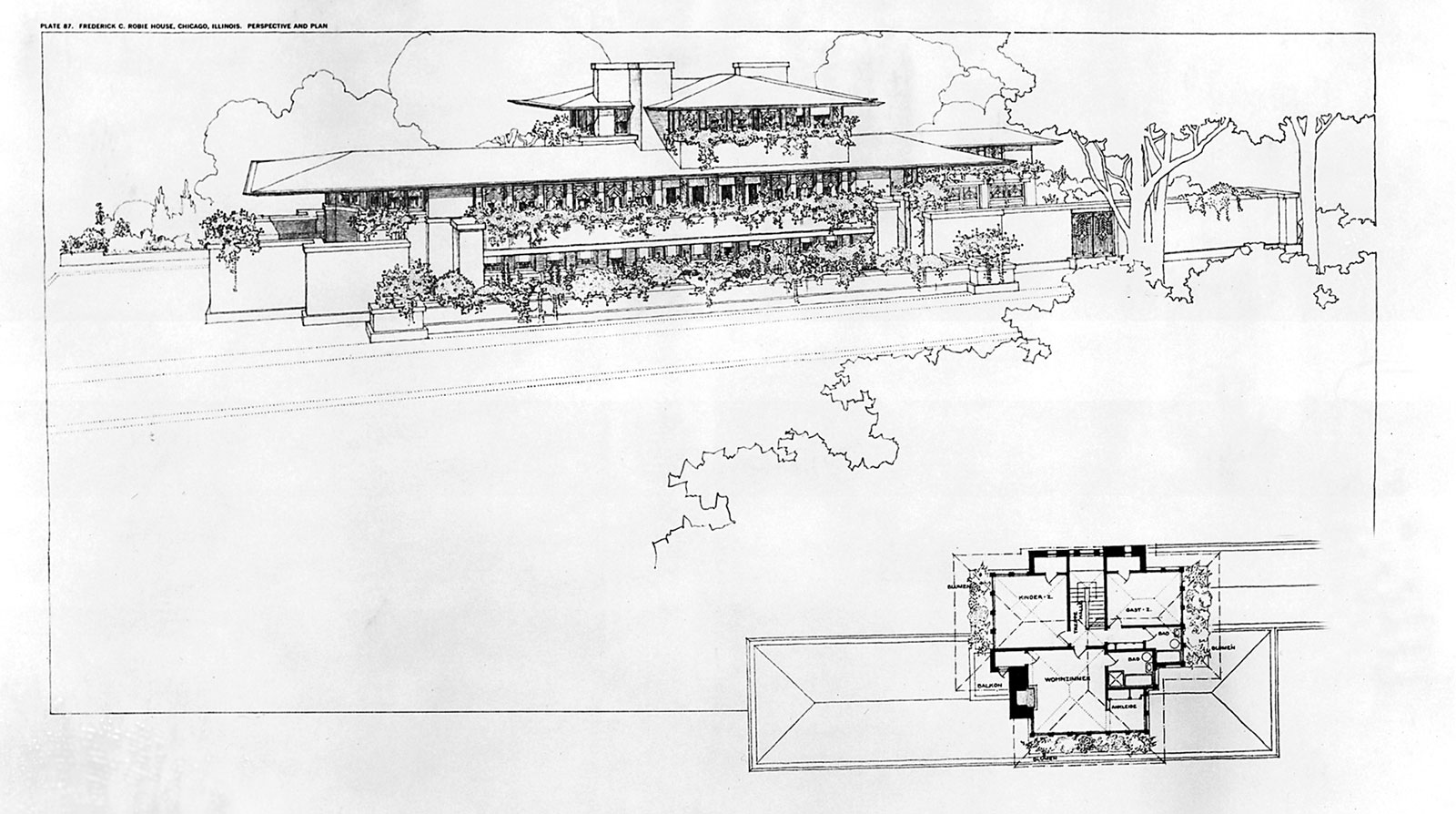This image is a detailed black and white architectural drawing titled "Plate by Frederick C. Robbie House, Chicago, Illinois: Perspective and Plan." It features a rectangular, three-story building with a significantly smaller top story. The house's distinctive design includes roof paneling that extends well beyond the sides, providing ample shading below. Windows line the front of this expansive residence, while three chimneys rise from its roof. The exterior is adorned with numerous plants, shrubs, and hanging foliage, both surrounding the base and decorating the balconies. The drawing also incorporates artistic elements such as trees and clouds, giving a complete perspective of the envisioned setting. In the bottom right-hand corner, there's a separate section that provides a top-down blueprint view of the house, detailing its layout from an aerial perspective.